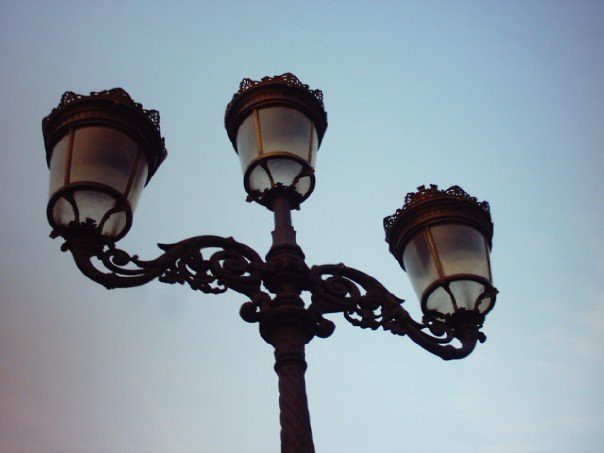In this outside photograph, an intricately designed, old-school lamppost stands prominently against a dim, possibly dusk sky. The sky is a mix of dark, dull blue with hints of clouds. The ornate lamppost is crafted from dark metal, likely black or dark brown, and features a twisted rope post that leads up to three large, cylindrical glass light fixtures, which are turned off. 

Each light is encased in glass with metal detailing, resembling crowns, adding to the lamp's elaborate design. The post branches into two arms that curve gracefully outward, reminiscent of open hands or scales, supporting the glass encasements on either side. A third light fixture sits atop the central rod, completing the trinity of lamps. The entire composition, with its intricate swirls and curves, suggests a vintage style, perfect for an old city park or historic urban area. The overall atmosphere of the image is dark and somewhat hazy, enhancing the antique aura of the scene.